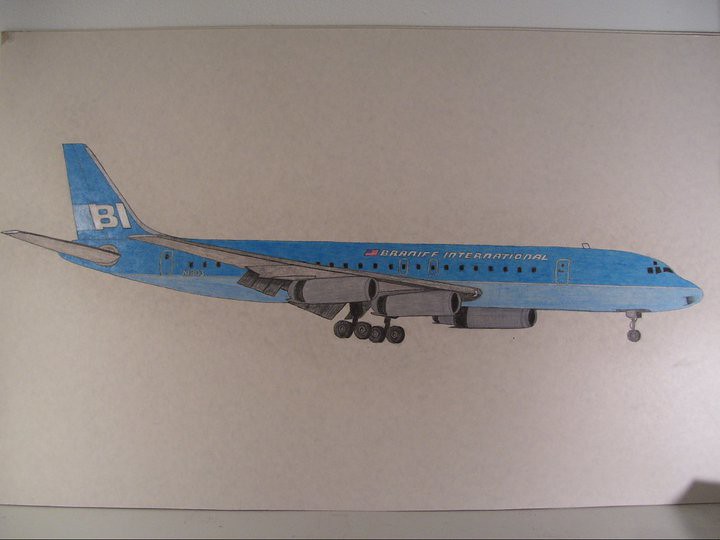This detailed illustration depicts a passenger airplane, resembling a 747 or 737, rendered in colored pencils or markers on a wide, landscape-oriented sheet of white paper, possibly from a sketch pad. The aircraft is characterized by its dark blue upper body and light blue lower body, with gray wings and engines. The tail features the initials "BI" in white. Centered on the fuselage, above a row of dark, rectangular windows, is the bold white text "Braniff International," accompanied by a small American flag. The landing gear is extended, with wheels visible, suggesting the plane is preparing for landing.